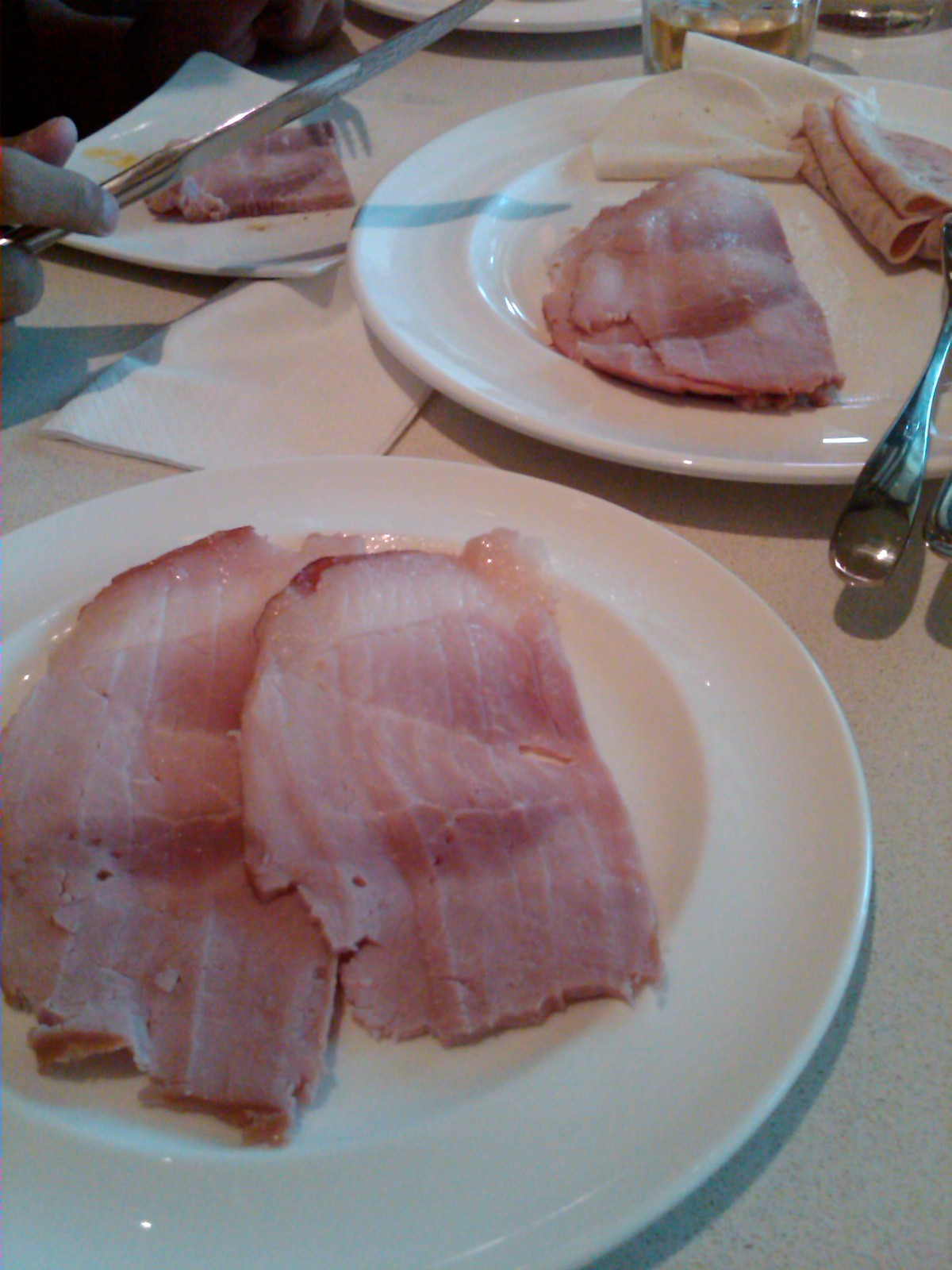This image captures a detailed table setting featuring multiple white plates with various breakfast meats. The closest plate, positioned at the front, contains two slices of what appears to be wide, striated bacon or thinly sliced ham. The second, slightly further back plate, also showcases similar meat along with some additional cold cuts and thinly sliced cheese, accompanied by a fork. Behind this plate, a glass of amber liquid, likely whiskey, is visible. To the left of the upper plate, a third plate shows only meat, possibly ham or turkey. Additionally, there is a partial view of a hand holding a knife near the left side of the image, showing two fingers and a thumb. The table surface is white, adorned with napkins, creating a simple yet organized dining scene.